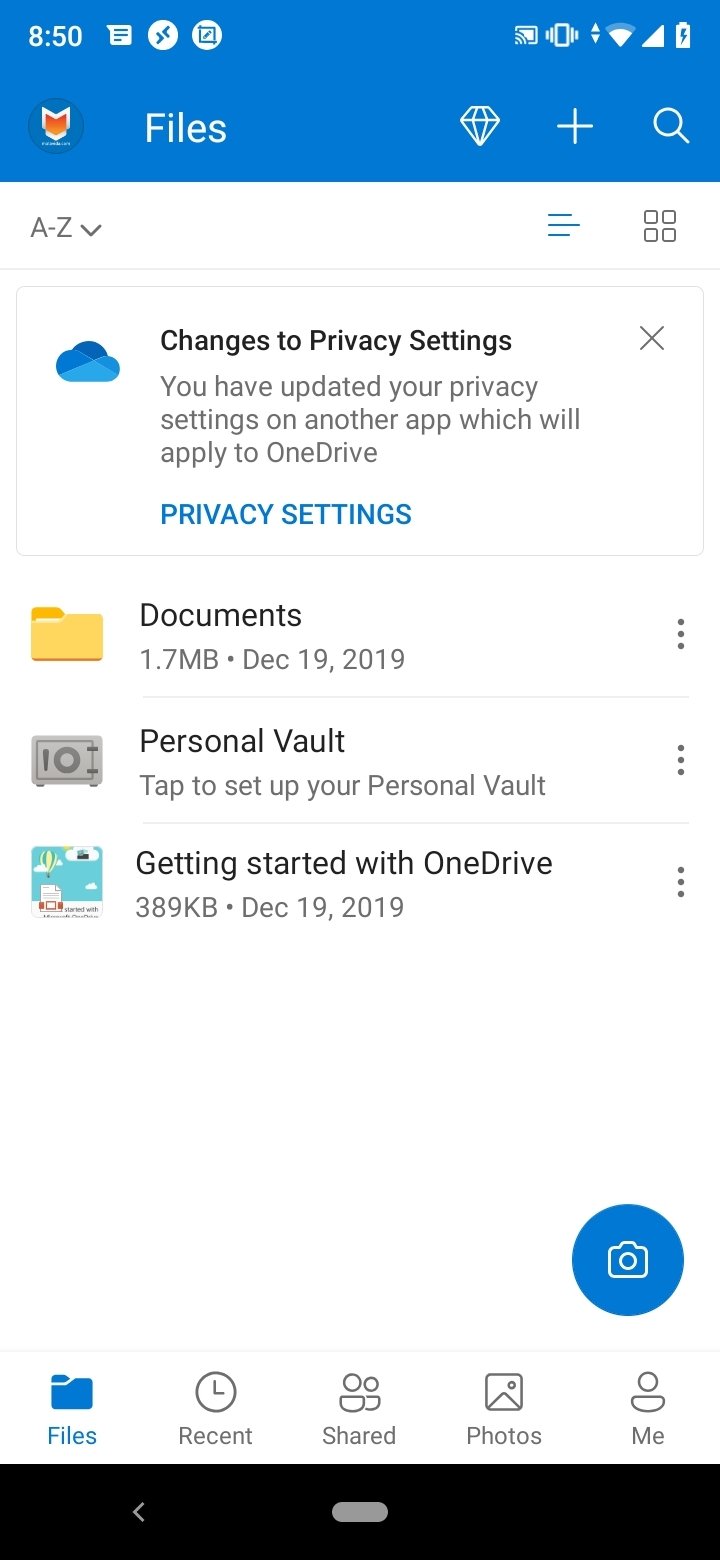This is a highly detailed and descriptive caption for the screenshot photo you provided:

---

A screenshot in portrait mode displaying a mobile phone interface, likely taken from an app managing files like OneDrive. The interface begins with a light blue header section comprising two rows. On the upper left-hand corner, there is a numerical value '850', and on the upper right-hand corner, a fully charged battery icon is visible.

Directly underneath, there's an icon resembling a red fox followed by the word 'Files'. Next to it, there are a diamond, a '+' sign, and a search icon aligned in sequence. Below this section, the background transitions to white.

The first row of the white section contains icons for 'A to Z', a down arrow, three lines, and a subsequent section. The prominent element in the next large block of text displays a message: 'Change changes to privacy settings. You have updated your privacy settings on another app which will apply to OneDrive.' On the right, there's an 'X', and on the left, the OneDrive cloud logo is visible, along with a blue 'Privacy Settings' link.

Following this, there is a row labeled 'Documents' paired with a folder icon, showing a file size of 1.7 MB and a date of December 19, 2019. The next row is 'Personal Vault' with a prompt to set it up. Below this, another row shows 'Getting started with OneDrive', 9 kilobytes in size, also dated December 19, 2019. Each entry in these sections has an accompanying 'three dots' icon for additional options.

At the bottom of this white area, it transitions to a section with a large blue circle containing a camera icon, indicating an application. Below, there are tabs labeled 'Files', 'Recent', 'Shares', 'Photos', and 'Me' with 'Files' being highlighted in blue. The entire interface is capped off by a black stripe at the very bottom.